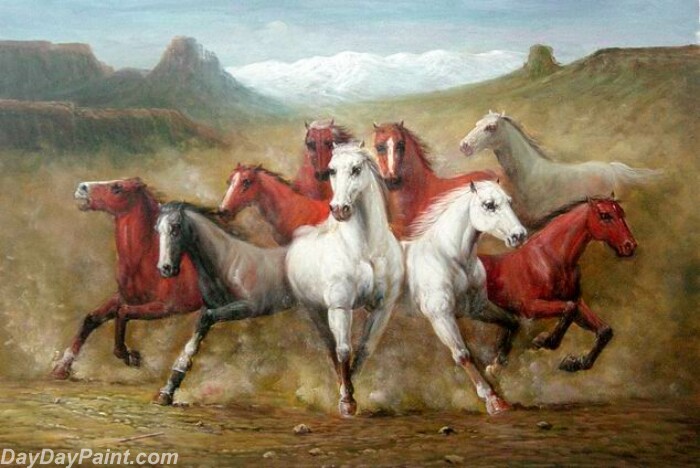The image features a vivid painting, likely created with colored pencils, depicting a dynamic scene of nine horses running through a dusty valley scattered with rocks and dirt, devoid of grass. The sky above transitions from white clouds to a blue expanse, and distant green and brown mountains form the backdrop. Prominently, the horses kick up dust as they run; three of them are white, one is brown, one is dark gray, and the remaining five are a reddish-brown color. Two of the reddish-brown horses have distinctive white stripes between their eyes. The painting is signed with "DayDayPaint.com" in the bottom left-hand corner.